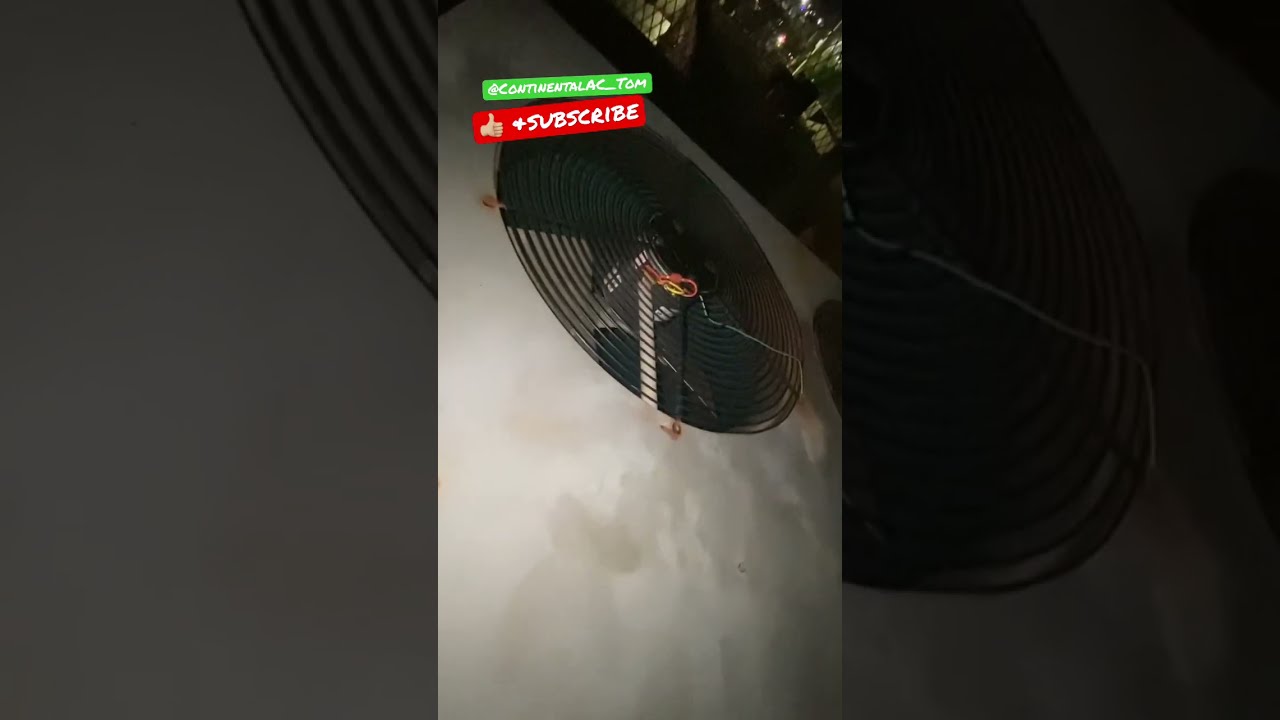The image prominently features an industrial-looking black fan situated in the center against a gray wall. The fan appears somewhat aged and rusty, with visible red, yellow, and blue wires extending from it. A protective circular grate covers the fan blades to prevent injury. Above the fan, there is a green banner with white text that reads "Continental AC Tom," likely a logo. Just below this banner is a red banner displaying a thumbs-up icon and the words "plus subscribe" in white. The composition suggests that the image might be part of an instructional video or TikTok format, possibly aimed at guiding viewers on air conditioning maintenance or repair. The background features a larger, blurred representation of the same fan, adding depth to the setup. The image combines various colors, including black, gray, red, yellow, blue, green, and white, displayed in a vertical format reminiscent of iPhone videos or social media content.